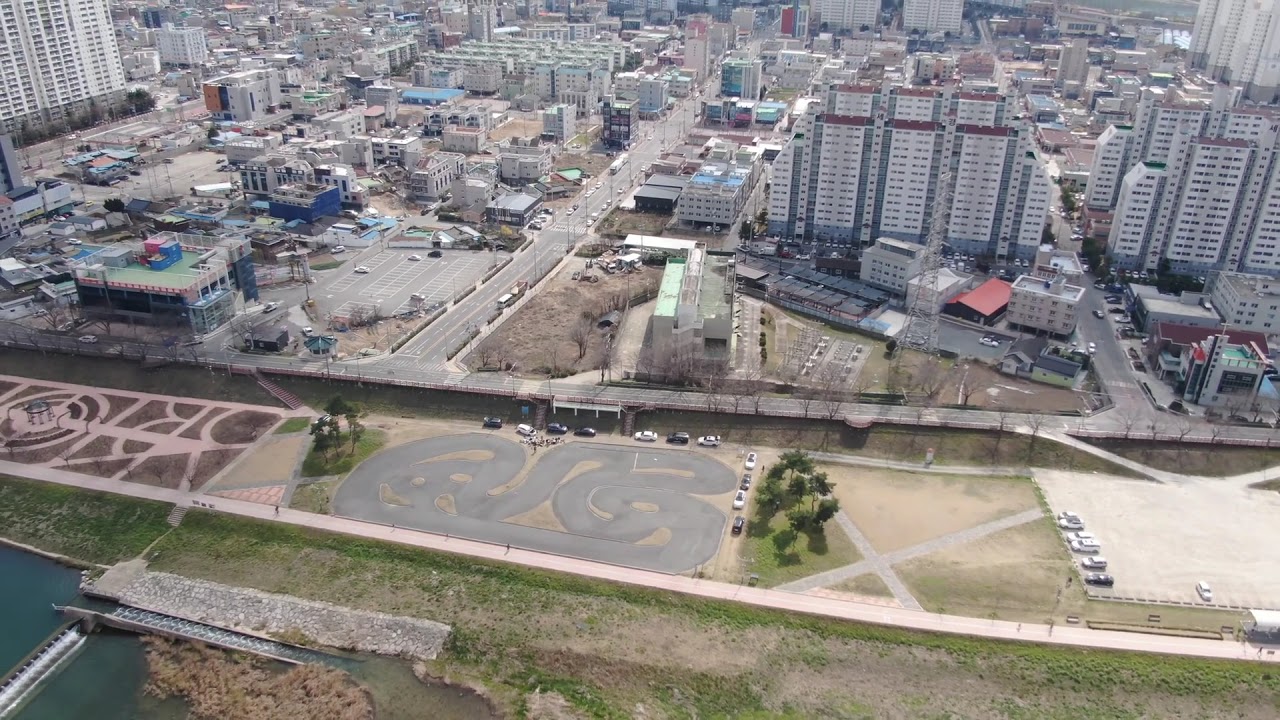This aerial photograph captures a daytime view of a cityscape with a rich blend of features. At the bottom left, a narrow canal or potentially a dam is visible, bordered by a grassy embankment. Above the embankment, a paved walkway stretches horizontally across the image, dotted with people taking advantage of the open space. To the right of this walkway lies a large parking lot with a few scattered cars and adjacent grassy areas, possibly gardens or parkways, adding a touch of green to the scene.

Centrally, a go-kart track or a repurposed recreational space can be seen, with cement paths that might be used for skateboarding or bicycling winding through it. Surrounding this area, you can spot additional green patches, particularly interestingly patterned gardens. 

Dominating the upper half of the photograph is the bustling city. The cityscape is densely packed with an array of buildings, ranging from tall white skyscrapers that resemble hospitals to smaller, varied structures. The streets, which appear parallel to each other, carve through the urban landscape, which is largely characterized by brown pavement and industrial features. This tightly packed area gives off an impression of being cramped and somewhat uninviting, lacking natural greenery but filled with the white and grey hues of modern architecture.